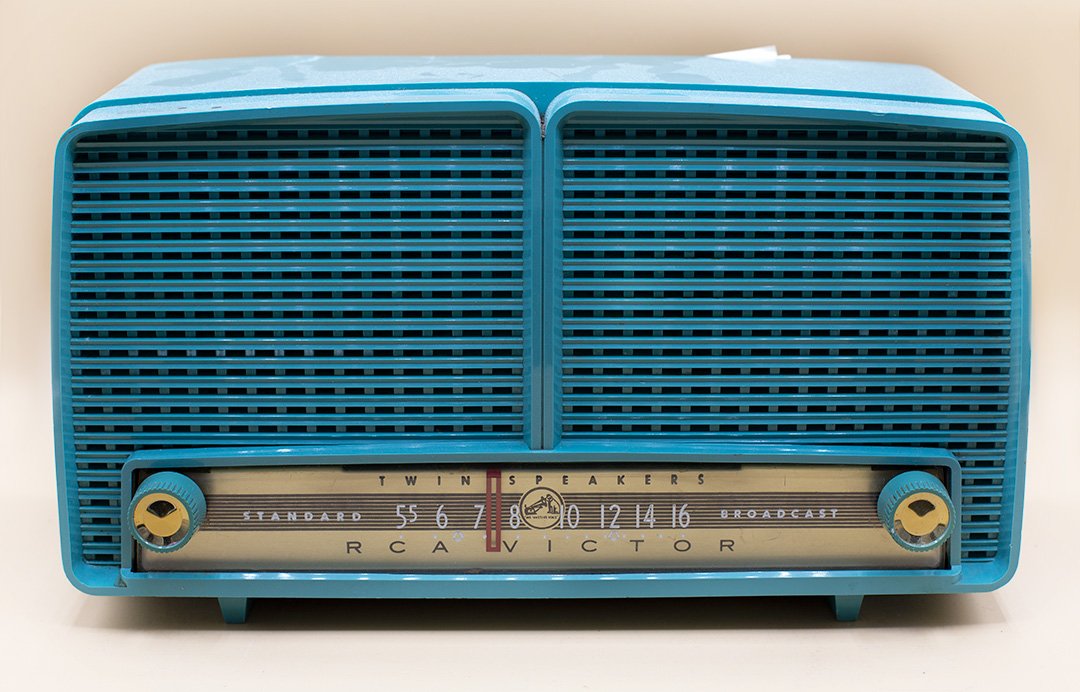This image depicts a vintage RCA Victor radio, characterized by its vibrant light blue plastic body and a rectangular shape. Prominently featuring twin speakers framed by a screen-like mesh on the front, the radio also showcases two silver and brown-topped dials on each side of the speaker array. The dials, set against a brown background, are located to the left and right of the station numbers, which range from 5 to 16, indicating standard broadcasting frequencies of that era. Below the dials, the words "twin speakers" and "standard broadcast 5567810121416" are inscribed, underscoring its classic design and functionality. Additionally, the maker's name, RCA Victor, is prominently displayed on the lower section, confirming its notable vintage craftsmanship. The radio rests on short, sturdy legs, adding to its retro aesthetic.